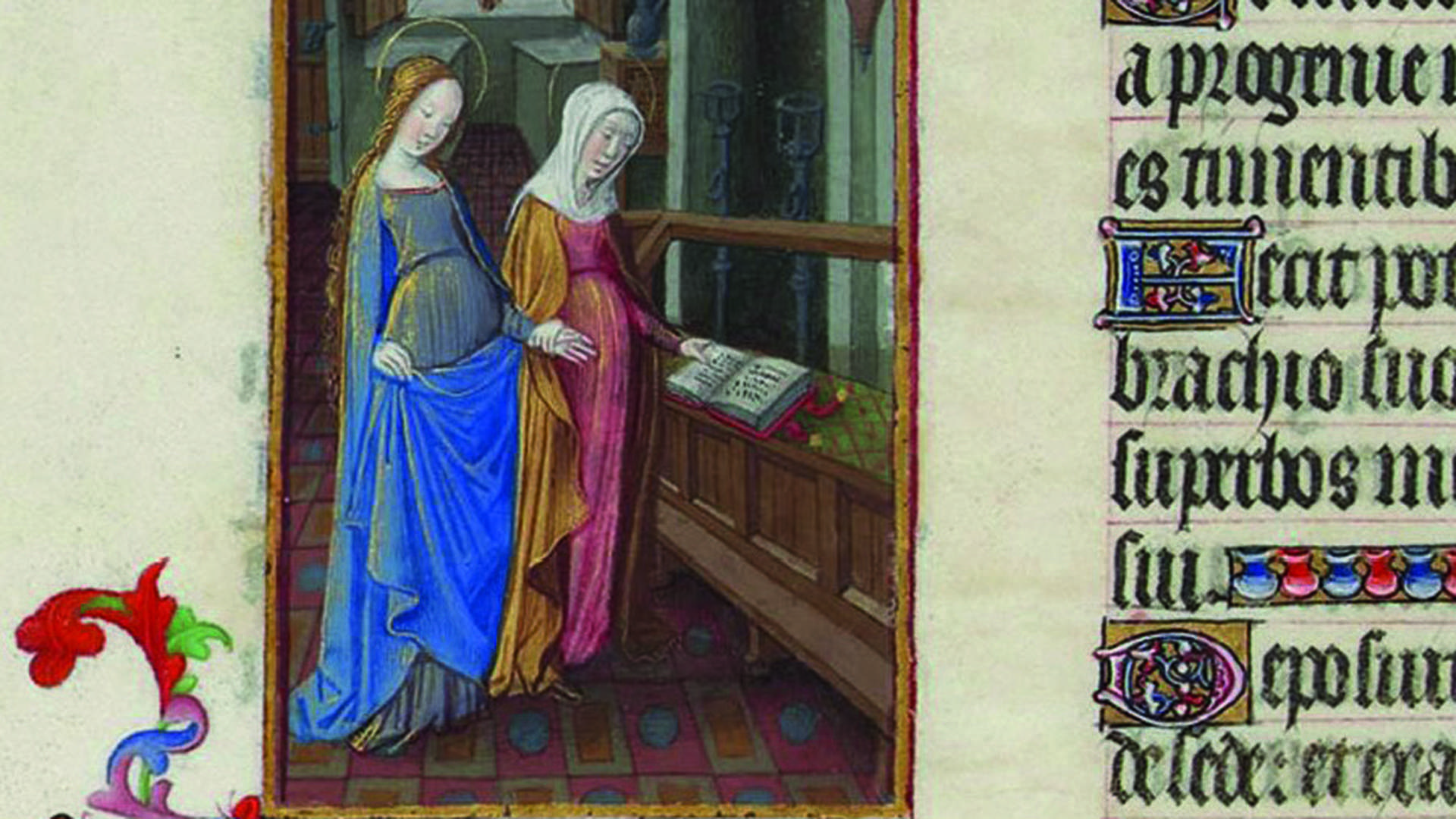This is a photograph capturing an old-fashioned, hand-drawn illustration steeped in a biblical ambiance. The centerpiece features two women, seemingly pregnant, adorned in long, flowing gowns reminiscent of sacred figures. The woman on the left wears a series of blues with a dark orange headpiece extending to the floor, while the woman on the right is dressed in a pink gown, complemented by an orange robe and a red head shawl. Both women, with halos above their heads, are immersed in reading a book placed on a wooden countertop. The backdrop suggests they are inside a house or possibly a church, with two unlit lanterns behind the book and a patterned floor of squares and circles, potentially signifying carpet or stone. To the far right, there is a column of text written in a language that resembles Old English or possibly Hebrew.